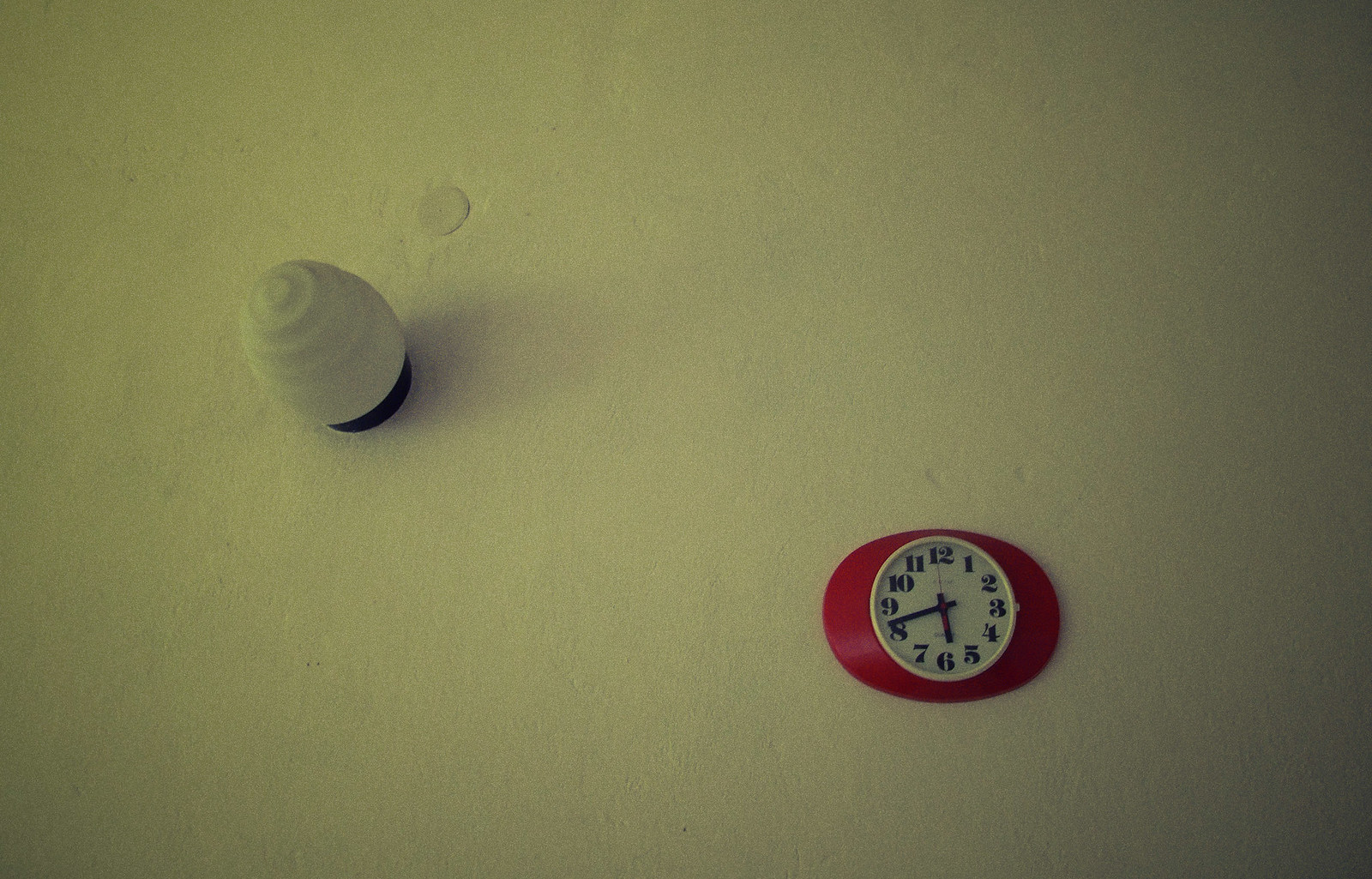This photograph captures a dimly lit mall, situated in a twilight setting, likely either dawn or dusk, given the subdued natural light. The walls of the mall are painted in a white or off-white hue. A striking red clock, displaying the time as 5:42, is prominently mounted on the wall. The clock features a white face with black or possibly navy blue hands, accented with a touch of red. Additionally, an unusual, swirl-shaped object, resembling an ice cream cone but possibly a light source or sensor, juts out from the wall. A circular plaster decoration is also visible on the wall, adding to the scene's intricate details.